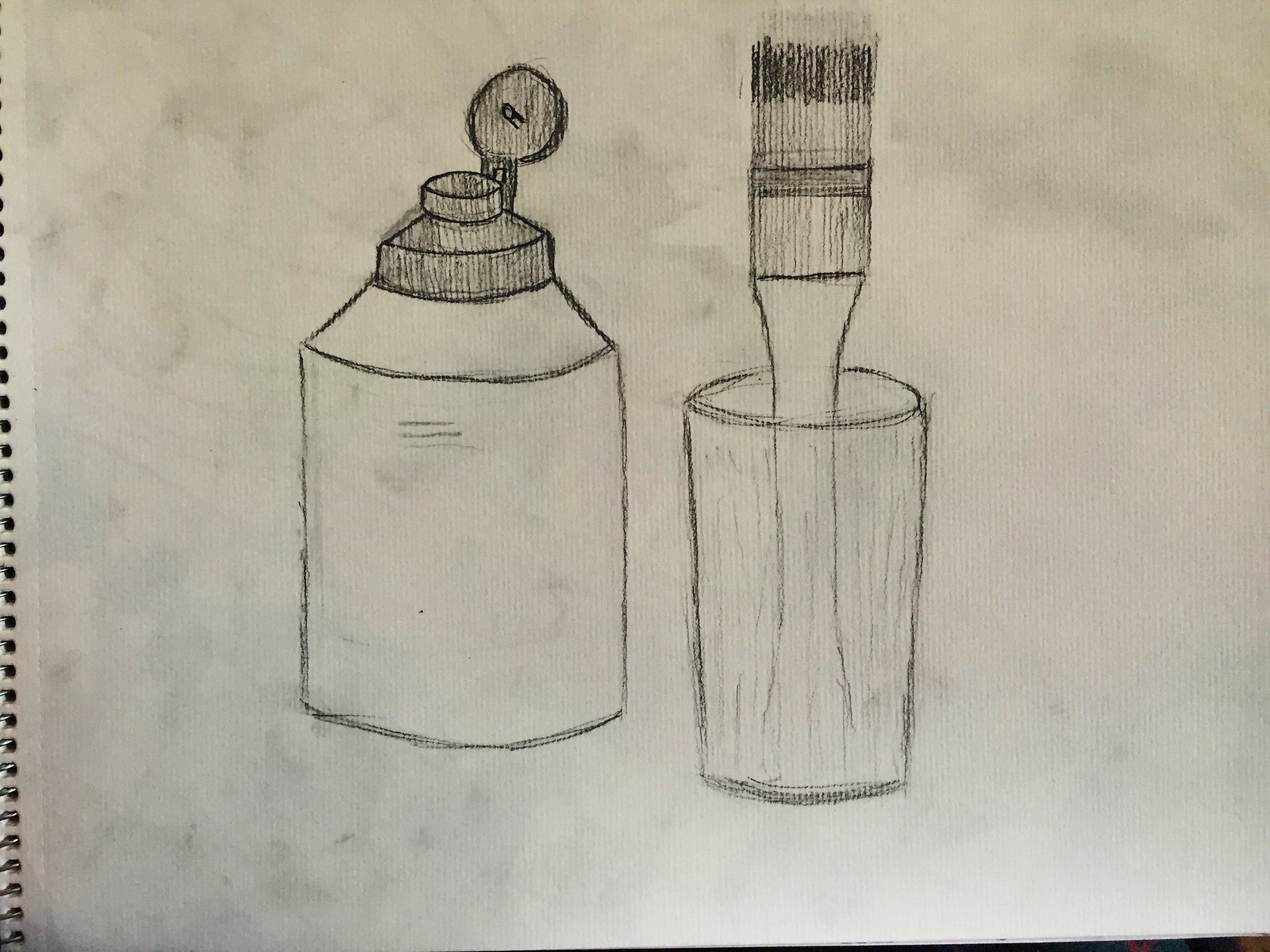This detailed caption synthesizes all the provided information:

The image depicts a detailed black and white pencil drawing on a slightly stained piece of notebook paper, identifiable by its perforated edge and ring holes on the left side. Dark shaded spots and splotches are visible across the paper, likely caused by the artist's hand smudging the pencil marks. On the left side of the drawing, there is a jar with a wood cap, wide at the base and tapering towards the top. The cap appears to be either shaded or textured with dark pencil lines. To the right, there is a simple round cup with a wide-headed paintbrush standing upright inside it. The brush is particularly detailed: its bristles are shaded, transitioning from light gray at the base to dark gray at the tips, suggesting it is laden with paint. The intentional shadowing and line work throughout the drawing give it a three-dimensional effect, emphasizing the textural contrast between the objects and the background.